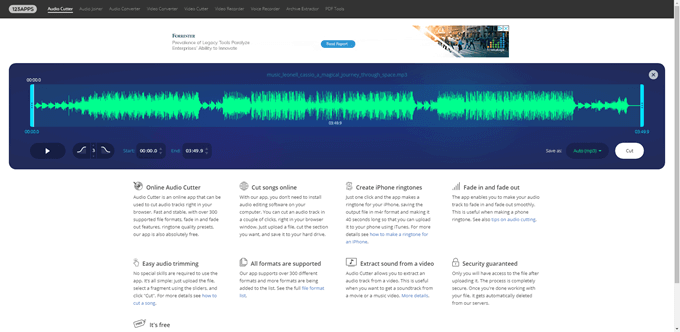A detailed screenshot of a music-producing application is prominently displayed. Dominating the center of the screen is a large blue rectangle symbolizing the main workspace, featuring a dynamic green line that represents sound waves. The width of the line varies—wider in some parts and thinner in others—indicating different sound amplitudes. Below this sound wave display are several smaller buttons for various functionalities, with the last button on the right being white and labeled "Cut."

In the upper right-hand corner of the rectangle, a small circle with an 'X' icon offers a quick option to close the workspace.

Further down, the interface divides into two rows, each containing four text boxes with headings: "Online Audio Cutter," "Cut Songs Online," "Create iPhone Ringtones," "Fade In and Fade Out," "Easy Audio Trimming," "All Formats Are Supported," "Extract Sound from a Video," and "Security Guaranteed." These headings likely indicate different features and capabilities of the application.

Finally, at the very bottom of the screen, there's a reassuring message indicating that the service is free, accompanied by a small price tag icon.